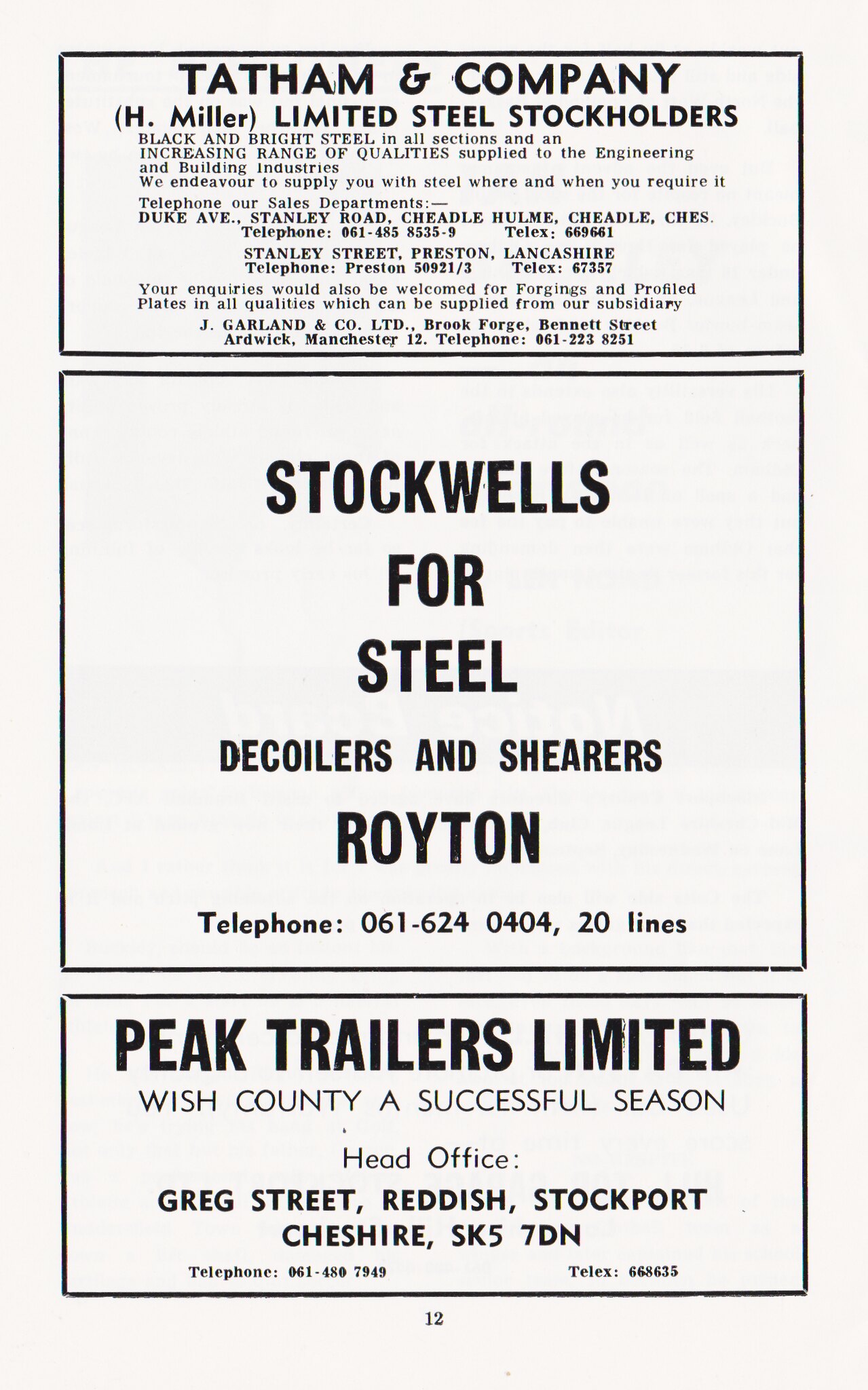This image features an old newspaper page, notably marked as page 12 at the bottom, which is entirely composed of advertisements from three different companies. The top rectangular ad with a black border showcases "Tatham & Company" in bold black letters. Beneath that, it states "H. Miller Limited Steel Stockholders" and advertises the availability of black and bright steel in various qualities for the engineering and building industries. 

The middle, and largest ad, belongs to Stockwells, proclaiming "For Steel, Decoilers & Shearers," with additional information: "Royton" and a contact number "061-624-0404" centered within the box.

The bottom rectangular ad, also framed with a black border, promotes "Peak Trailers Limited" with the message, "Wish County a successful season," followed by the office address: "Greg Street, Reddish, Stockport, Cheshire, SK57DN."